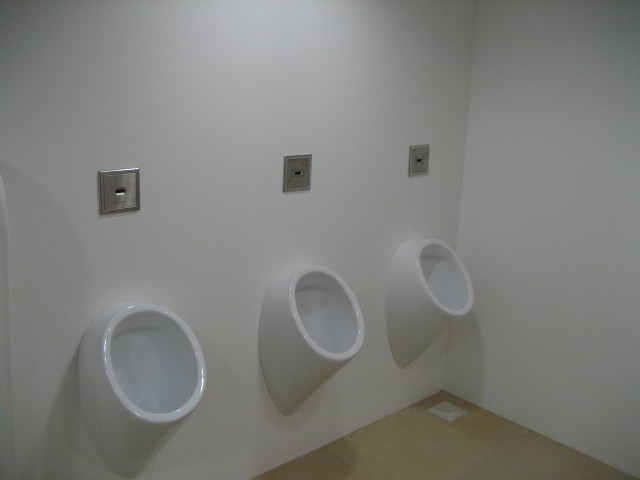The image depicts an indoor men's restroom with three, well-polished, white porcelain urinals mounted against a white wall. These urinals are small, circular bowls that are angled steeply from the wall. Above each urinal, there are square, metal sensors which are infrared detectors that facilitate automated flushing. The floor is covered in light brown tiles. At the bottom right corner, beneath the urinal on the far right, there is a small white disc on the floor, along with a white square, adding subtle detail to the setting. Additionally, light from an unseen source illuminates the upper part of the wall, reflecting softly, enhancing the clean and straightforward ambiance of the restroom.